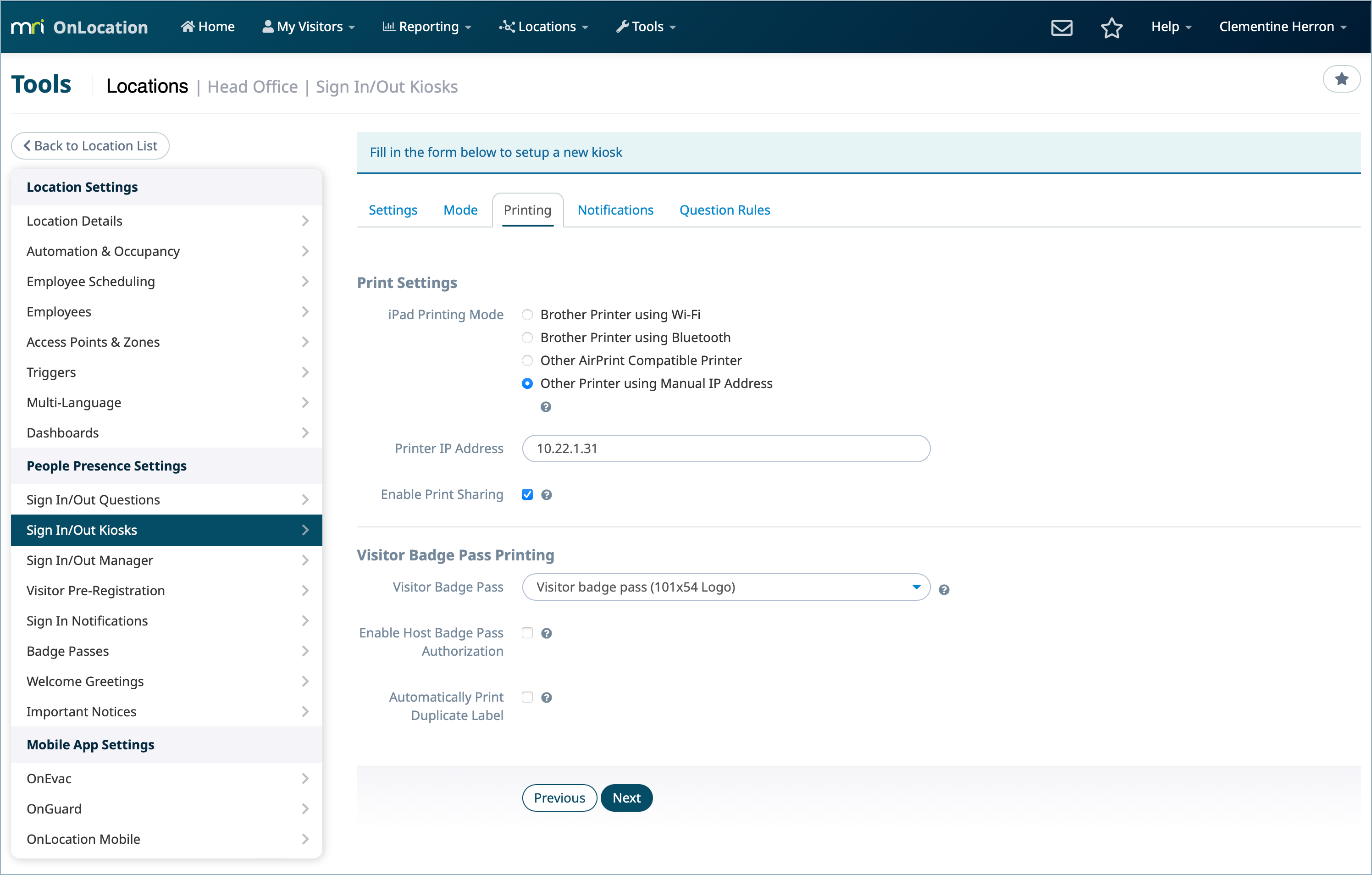The image showcases a detailed view of a website interface belonging to 'MN Tools.' The primary navigation bar at the top features several options including 'Home,' 'My Visitors,' 'Repairing Locations,' 'Tools,' and a 'Help' link on the right. Accompanying these are two icons and a text label reading 'Clementine Heron.'

Alongside the 'Tools' tab, other listed sections include 'Locations,' 'Head Office,' 'Sign In/Out,' and 'Class Kiosks.' Additionally, there is an option to return to the 'Location List' and access 'Location Settings.'

On the left-hand side of the website's body, users are prompted with "Fill in the form below to set up a new kiosk." Below this prompt are several highlighted and clickable options including 'Settings,' 'Mode,' 'Pricing,' 'Notifications,' 'Question Rules,' and 'Print Settings.' In the 'Print Settings' section, 'Printing Mode' is a highlighted term.

Within the 'Printing Mode' sub-menu, options include 'Other Printer Using Manual IP Address,' with an accompanying checkbox for 'Enable Print Sharing.' The 'Visitors Badge Pass' feature is prominently highlighted. Beneath it are further options to 'Enable Host Badge Pass' and 'Automatically Print.'

At the bottom of the form, navigation buttons are presented with a white 'Previous' button on the left and a blue 'Next' button on the right.